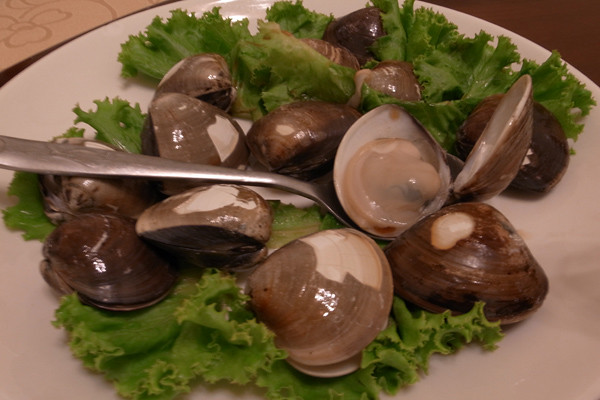This close-up image showcases a circular white plate adorned with a bed of vibrant green romaine lettuce leaves. Atop the lettuce, there are approximately seven to eight clams, with their closed, glistening shells varying in colors from light tan to dark brown, and some with white markings. One clam, positioned centrally on a spoon, is open, revealing its light beige interior, which somewhat resembles a human tongue. The plate's background edges capture hints of a tablecloth with a patterned design in the upper left corner and a dark brown area in the upper right, suggesting a table beneath it. The detailed arrangement highlights the freshness and presentation of the clams on the plate.